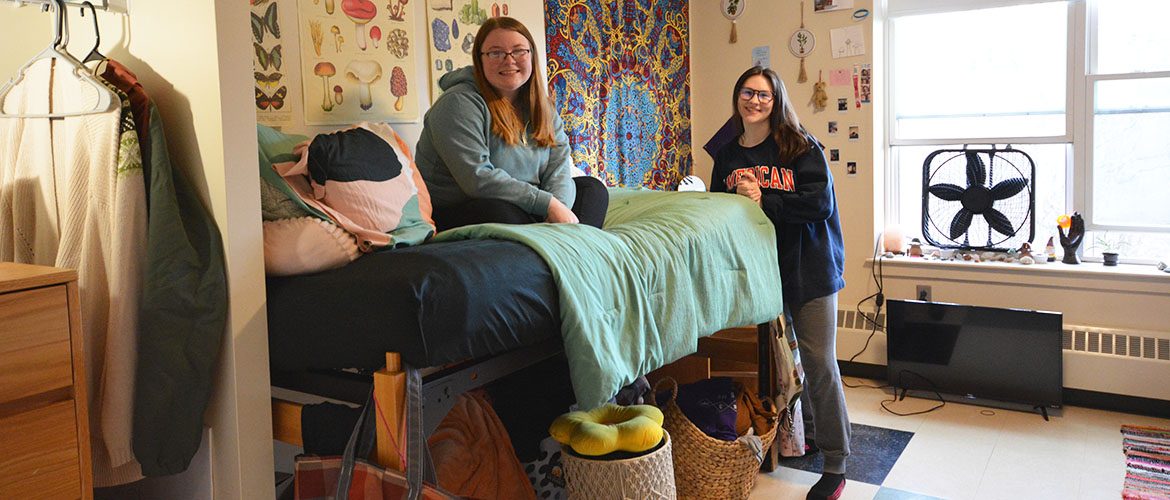This detailed photograph captures an indoor college dorm room setting, taken from the viewpoint of someone standing at the doorway. The main subjects are two young women, both of Caucasian descent and wearing glasses, positioned centrally in the image.

On the left side, a woman with long reddish-brown hair parted at the side is sitting cross-legged on a high bed elevated by black metal risers. She is dressed in a green hoodie and dark pants, with a green blanket and pink pillows visible on the bed. Behind her, the wall is adorned with various posters depicting butterflies, mushrooms, and rocks. There are also decorative blankets and suncatchers hanging on the wall.

To the right of her stands another woman with long brown hair parted in the center. She is wearing a blue sweatshirt with partially obscured red and white text that likely spells "American," along with gray pants. Her hands, positioned in front, obscure some of the lettering on her sweatshirt.

The room features tiled flooring, a large flat-screen TV placed on the floor in front of a heater register beneath two large windows, one of which has a window fan attached. Additional room details include a cut-off image of a brown two-drawer chest, some jackets and sweaters hanging from a rod to the left, and baskets stowed underneath the bed. The walls are painted beige and dotted with various stickers, contributing to the cozy and personalized atmosphere of this college dorm room.